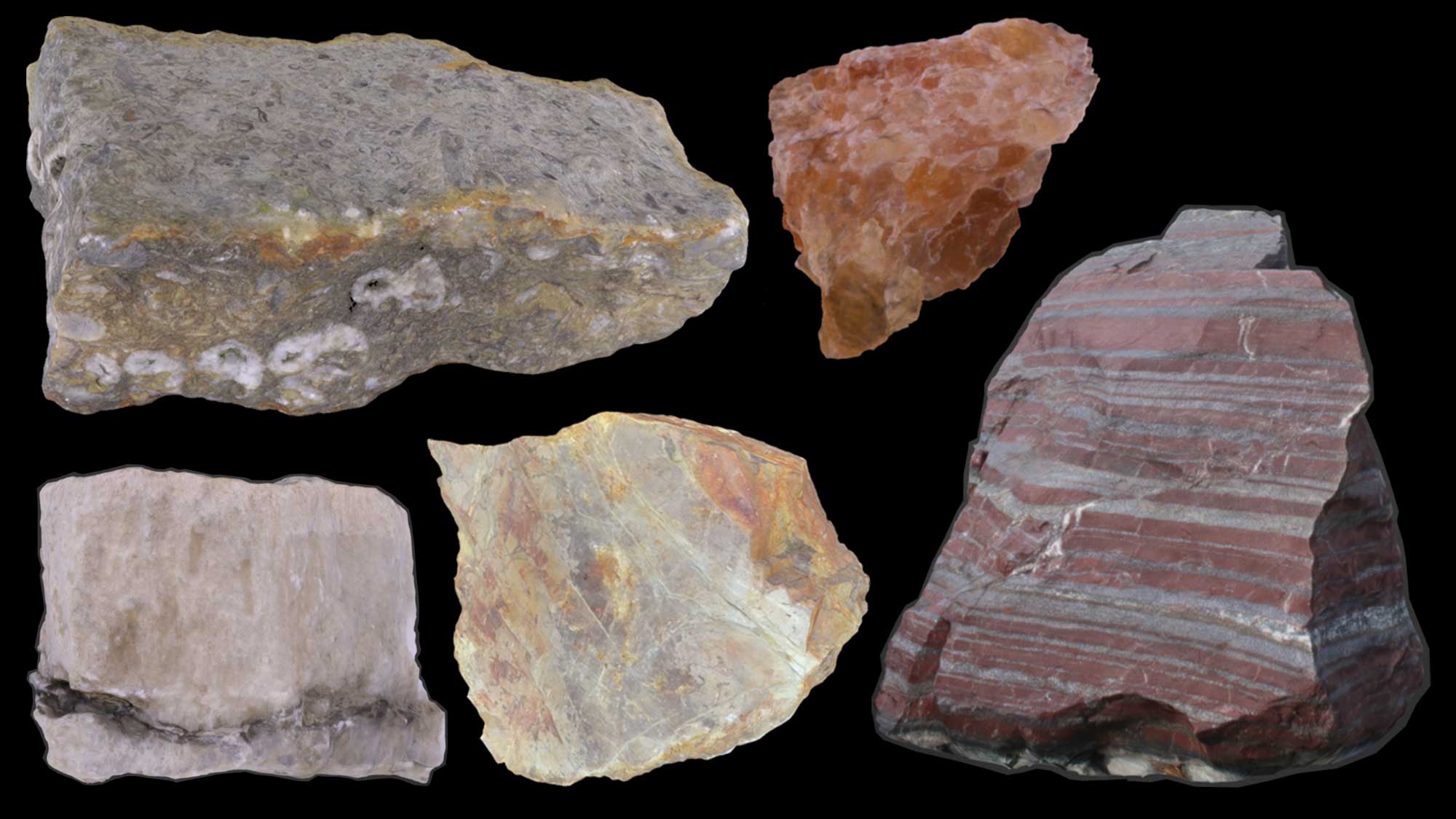The photograph showcases a striking assortment of five distinct minerals against a completely black background, which may give the impression of a museum display. The minerals are arranged thoughtfully, with two positioned at the top and three at the bottom. 

Starting from the top left, there is a gray rock with hints of yellow and white. Next to it is an orange-shaded mineral, adding a warm contrast to the cool tones around it. At the bottom right, a triangular-shaped rock catches the eye, its surface adorned with intricate grey and red lines.

In the center, a pale, limestone-like mineral with a calcium-rich appearance stands out, while to its right, a mineral with a smooth, grayish surface and layered texture reminiscent of basalt or granite adds to the diverse display. The array also includes a fascinating green mineral, crystalline in nature, which juxtaposes against another rocky mineral with a murky green tint. Together, they present a captivating spectrum of colors, textures, and geological curiosities.